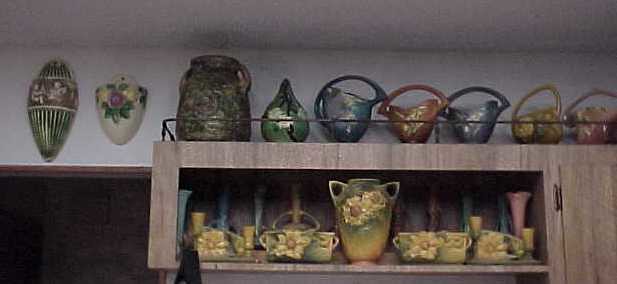The image displays various ceramic dishware arranged neatly on wooden shelves. The shelves are light brown and part of a cabinet where the door is barely visible in the right corner. On the top shelf, there are seven bowls in a sequence of colors: pink, yellow, blue, orange, blue, green, and green. In front of these bowls, there are four cups with yellow flower designs, placed two on each side of a prominent vase that also features yellow flowers.

Below this top shelf, two matching sets of floral-scented ceramic vessels can be seen, each adorned with intricate flower designs in green and yellow hues. Additionally, scattered across the shelves are various ceramic containers, vases, and vessels that vary in size and shape. Among them, several have a handle extending all the way across the top, adding to the variety of forms.

Above the shelving unit, just under the ceiling, there are two wall vases—one green and brown, the other white with pink and yellow flowers. Each piece of dishware exhibits muted colors, including shades of green, blue, yellow, orange, and pink, creating a harmonious and vibrant display of ceramic artistry.